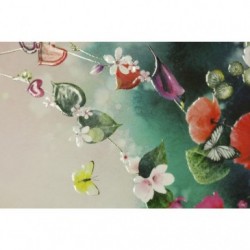The image is a small, close-up depiction that blurs the lines between a painting and a beaded artwork, possibly resembling elements of a greeting or Christmas card due to its intricate details. The background transitions from a light gray on the left to a mix of greens and darker blues on the right, giving it an ombre effect. At the center, a delicate green vine curves upward, adorned with a series of flowers and leaves. Among the floral elements are white, purple, and peach-colored flowers, interspersed with tiny white blossoms and green heart-shaped leaves. The flowers seem meticulous and almost bead-like, suggesting they could be part of a necklace, especially with a silver wire threading through the arrangement. There's a prominent yellow butterfly at the bottom with an embossed plastic glow, reflecting light. Another black and white butterfly with a larger wingspan is positioned near the top vine. Additional heart and flower-shaped beads in pink and other colors are scattered throughout the vine, creating a visually rich and dynamic composition against the nebulous blue to white background that adds to the ethereal beauty of the artwork.